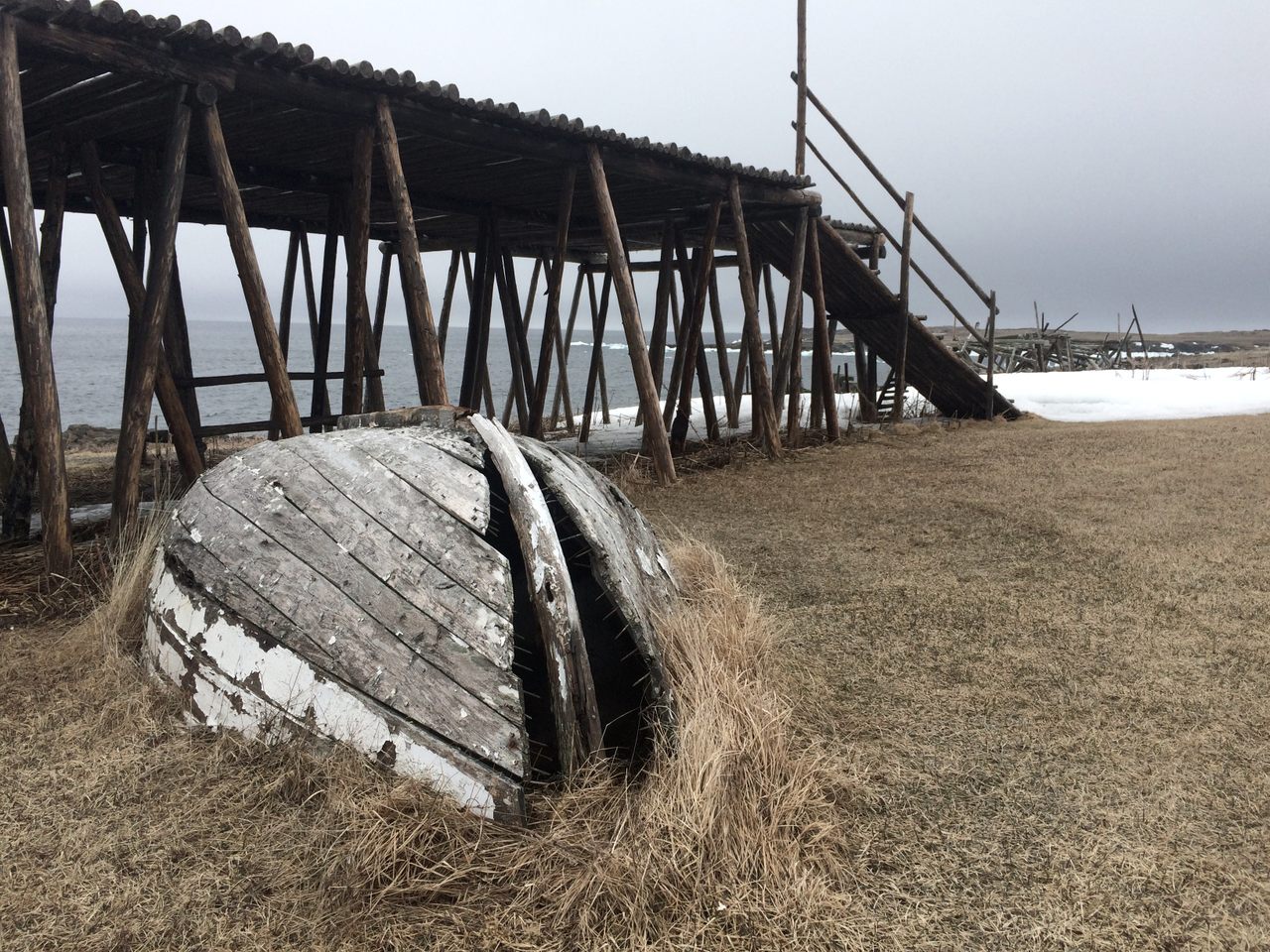This photograph captures a desolate, almost eerie scene of an old, wooden boat that has washed ashore and sits cracked open and abandoned on a field of grayish-brown grass. The boat, small and overturned, appears as though it has been neglected for a significant time, its wooden boards split and nails protruding, reminiscent of a cracked melon. To the left of the scene lies the sea, its grayish-blue waters meeting the horizon under an equally gray, dull sky, contributing to the somber atmosphere. In the top left corner, an elevated dock on wooden stilts extends over the grass, its wooden stairs leading down to a patch of white sand, suggesting proximity to a beach. Snow dusts the ground to the right, adding to the chill of the scene. Overall, the landscape feels desolate and off-putting, with no signs of human presence to bring warmth or life to the stark, watery area.